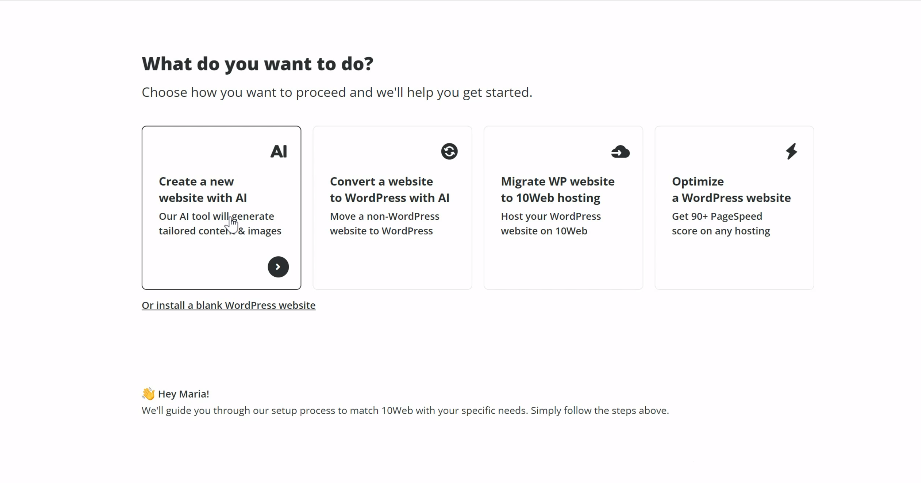The image appears to be a screenshot of a web page with a white background and predominantly black text, resembling the top section of an email or a website interface. On the top left corner, there is bold text that reads "What do you want to do?" with a subheading beneath it saying "Choose how you want to proceed and we'll help you get started."

Below this, there are four distinct options presented, each within its own bordered container. The first option on the left is highlighted and labeled with "AI" in its top right corner. It reads "Create a new website with AI: our AI tool will generate tailored content and images." The mouse pointer is hovering over this option, indicating it is currently selected.

The second option, which is located next to the first, says "Convert a website to WordPress with AI: move a non-WordPress website to WordPress." 

The third option is titled "Migrate WP website to 10Web hosting: host your WordPress website on 10Web." 

The fourth and final option reads "Optimize a WordPress website: get 90+ page speed score on any hosting."

Directly beneath these options, there is a clickable link that states, "Or install a blank WordPress website."

At the very bottom of the page, there is a yellow waving hand emoticon accompanied by the text, "Hey Maria, we'll guide you through our setup process to match 10Web with your specific needs. Simply follow the steps above."

The entire image conveys a clean, user-friendly interface designed to help users choose how they want to set up their WordPress website with the help of AI tools and other options provided by the platform.